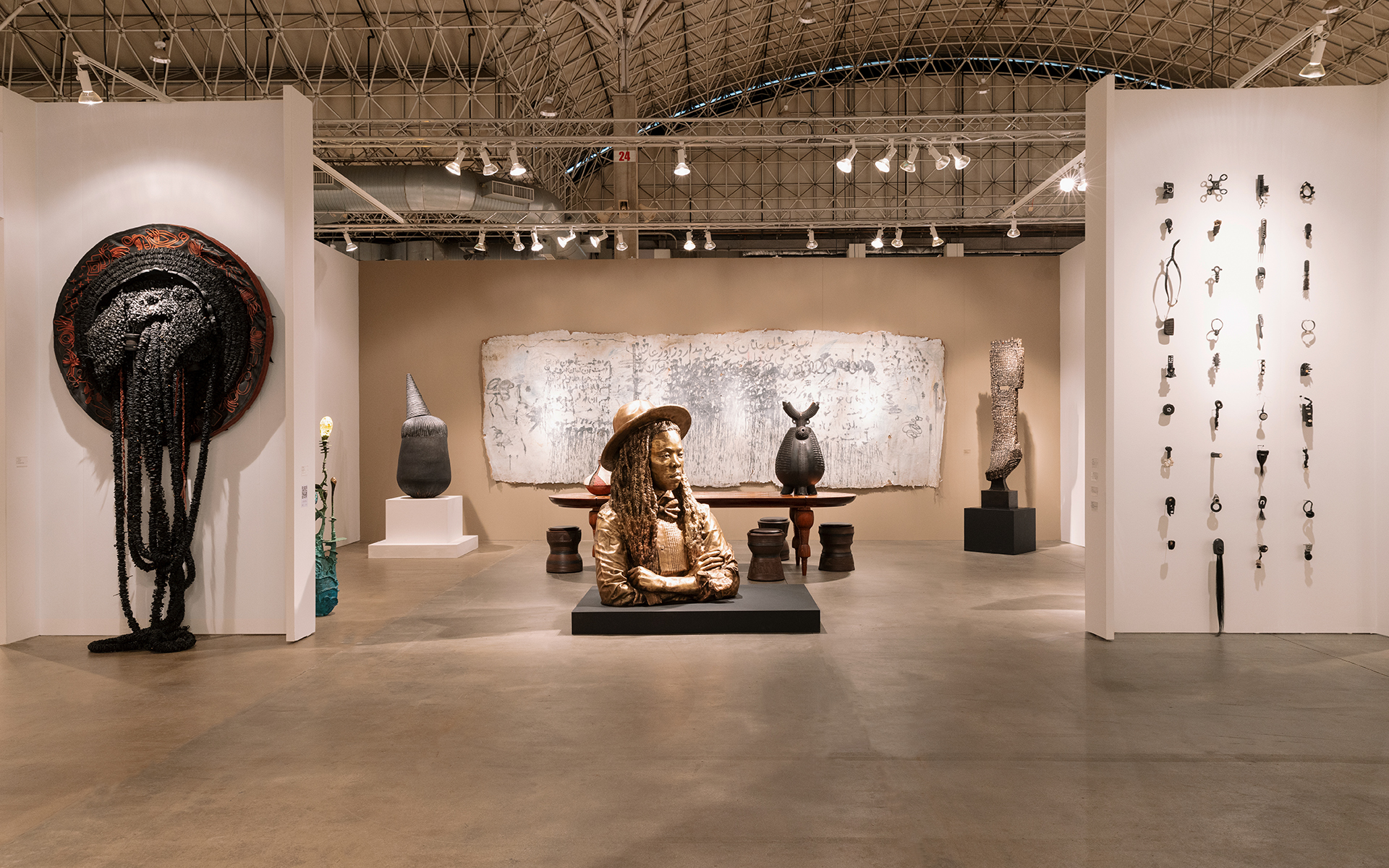This detailed interior shot captures an art exhibit or museum room with partial floating walls that don't reach the ceiling, supported by metal trusses with bright lights highlighting the artworks. At the center stands a striking bronze bust of a woman with long curly hair, wearing a broad-rimmed hat, scarf, and jacket with rolled-up sleeves; her serious expression suggests an African origin, aligning with the other African-themed pieces in the room. To her right, a wall displays a grid of objects resembling tools or hooks. Behind her is a table adorned with what appears to be a small carved kangaroo and four rounded chairs resembling chess pieces. On the left wall, there is a large circular piece with ropes or vines extending down to the floor. The back of the room features a large sculpture that could resemble a bone, and a simpler rounded-off shape with a pointed top. Against the far wall, a piece, possibly a painting or calligraphy, displays illegible writing, adding an intriguing, albeit mysterious, element to the exhibit.